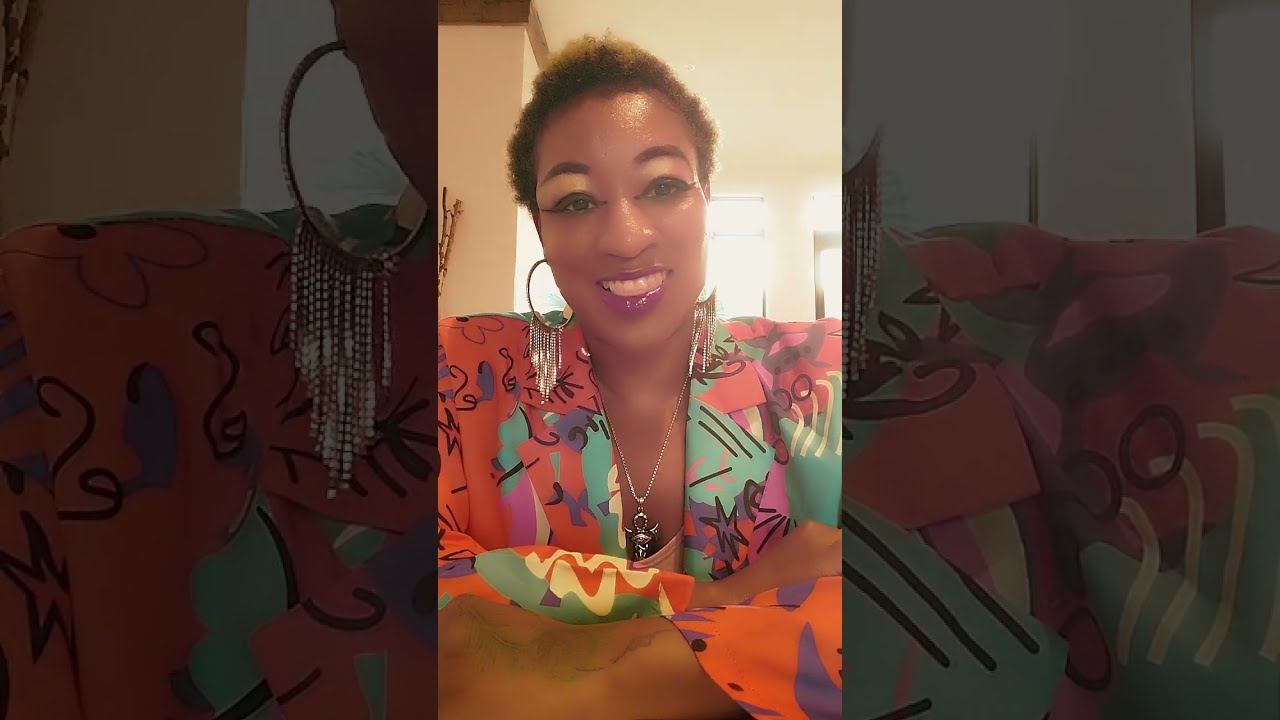The image showcases a smiling African-American woman, possibly in her 30s, with short hair, wearing extensive makeup. Her eyebrows feature a hint of gold, and her lips are adorned with purple lipstick. She has bright, expressive eyes highlighted by her makeup. Her attire is notably vivid, consisting of a multicolored suit filled with abstract patterns and a palette of green, red, orange, yellow, blue, and violet. Beneath the low-necked or v-necked blouse, she dons a necklace featuring a pendant that resembles an animal head or a character. She accessorizes with large hoop earrings that have a chandelier-like appearance. Her arms are crossed in front of her, revealing a hint of what appears to be a tattoo. The room she is in has white walls with brown trim, and sunlight streams in through a window, adding a warm glow to the scene. This primary photograph is further enhanced by a blown-up, dimmer version of the same image as the background, creating a layered visual effect.